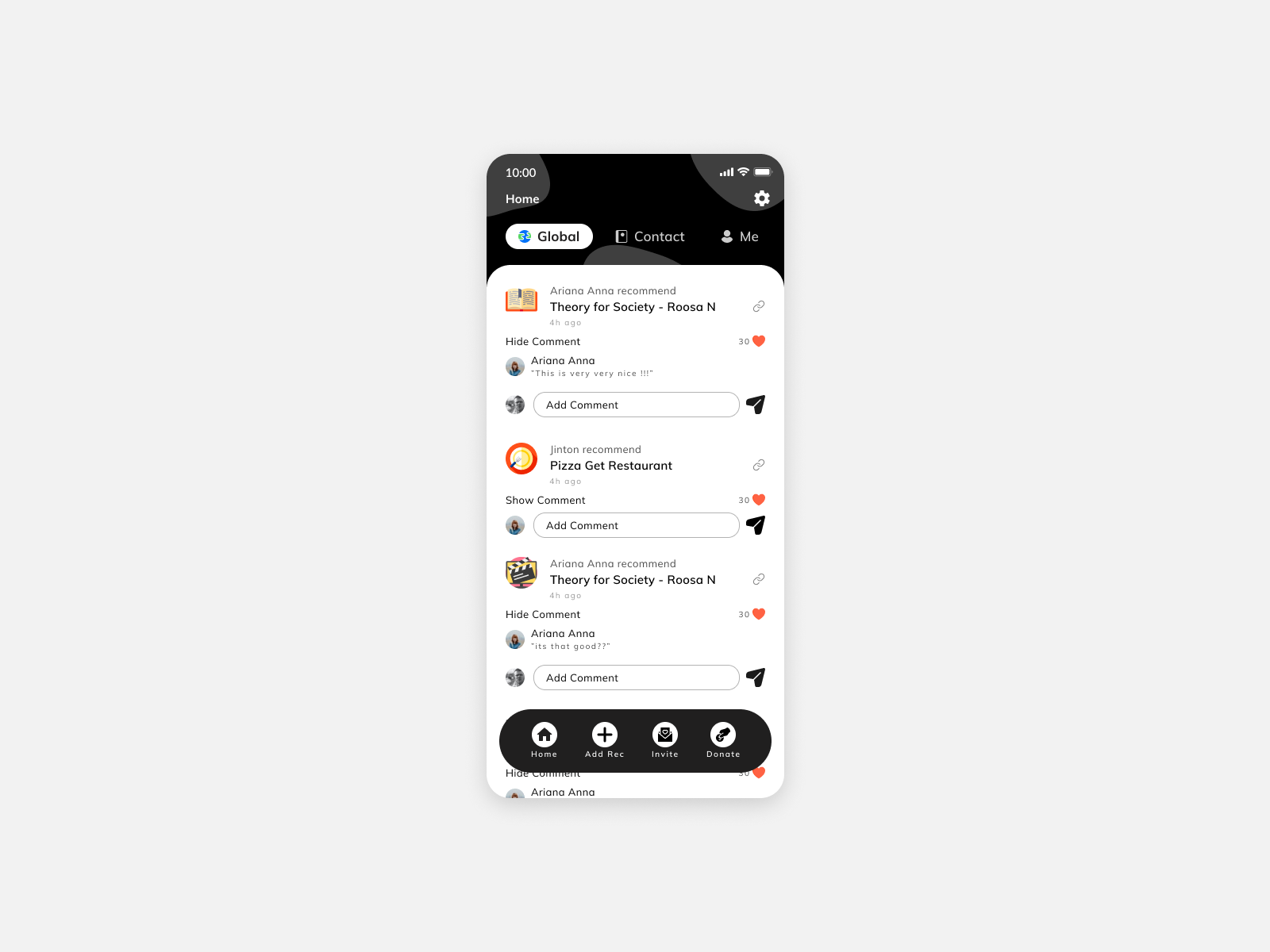Here is the cleaned-up and detailed caption for the screenshot image:

---

The screenshot captures a digital interface displayed primarily in light gray with a central focus on a phone screen. At the top left corner of the phone screen, the time is shown as 10:00, below which the word "Home" is displayed. The top right corner shows the internet connectivity bars, the battery level indicator, and a settings icon.

The top section of the interface has a black background adorned with gray blobs and features three categories: "Global" with a world icon (highlighted with a white background), "Contact," and "Me," both displayed with white text on a transparent background.

The major portion of the screen consists of text and interactive elements divided into sections. At the top, the text reads "Ariana and Ariana Anna recommend theory for society - Root Rosana," followed by "4h ago" in small text. To the right, there's an icon resembling a chain link, indicating a hyperlink, and an open book icon on the left. Below, a clickable option to "Hide comment" is visible.

Under this, an icon of a girl with red hair and a light complexion appears next to the name "Ariana." The comment states: "This is very, very nice!!!" To the right of this comment, a heart icon accompanied by the number "30" indicates likes or favorites. An "Add Comment" bar follows, with a picture of a man with dark hair to its left and a triangle pointing upward on the right.

Subsequently, the text reads "Jinton recommends Pizza Get Restaurant" followed by "4h ago." To the right is another chain link icon, and to the left, an icon resembling a pizza. Below, there is an option to "Show comment," an icon of the same girl with red hair, an "Add Comment" bar on the right, and a heart icon with the number "30."

Further down, there is another recommendation for "Theory for Society - Roosa," with a movie icon on the left. Beneath this, the text reads: "Hide comment Ariana" followed by the quote "It's that good??" To finish, there are four icons aligned horizontally above the text bar labeled "Home," "Add," "Rec" (indicating recording), "Invite," and "Donate."

---